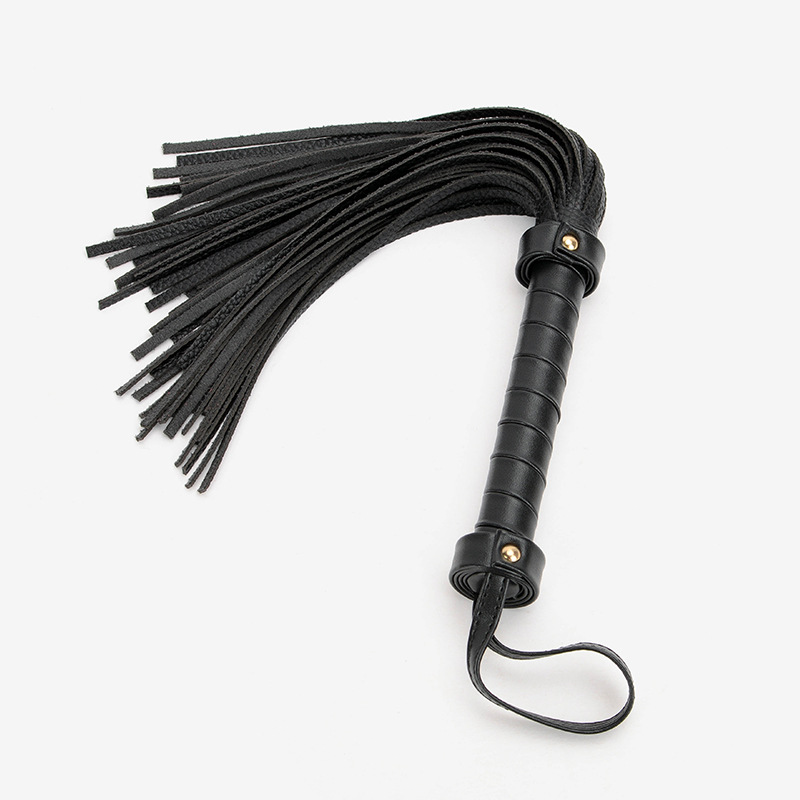The image is a digital photograph featuring a single black leather flogging whip placed on a white background. The whip appears to be in brand new condition. Its handle is adorned with brass or gold-colored pins that secure the top and bottom parts, enhancing its aesthetic appeal. The handle ends with a keychain-like hook, made from the same black leather, designed for hanging. Multiple lashes extend from the top of the whip, emphasizing its purpose. There is no text in the image, which focuses solely on the detailed craftsmanship and contrasting colors of black leather and brass elements.